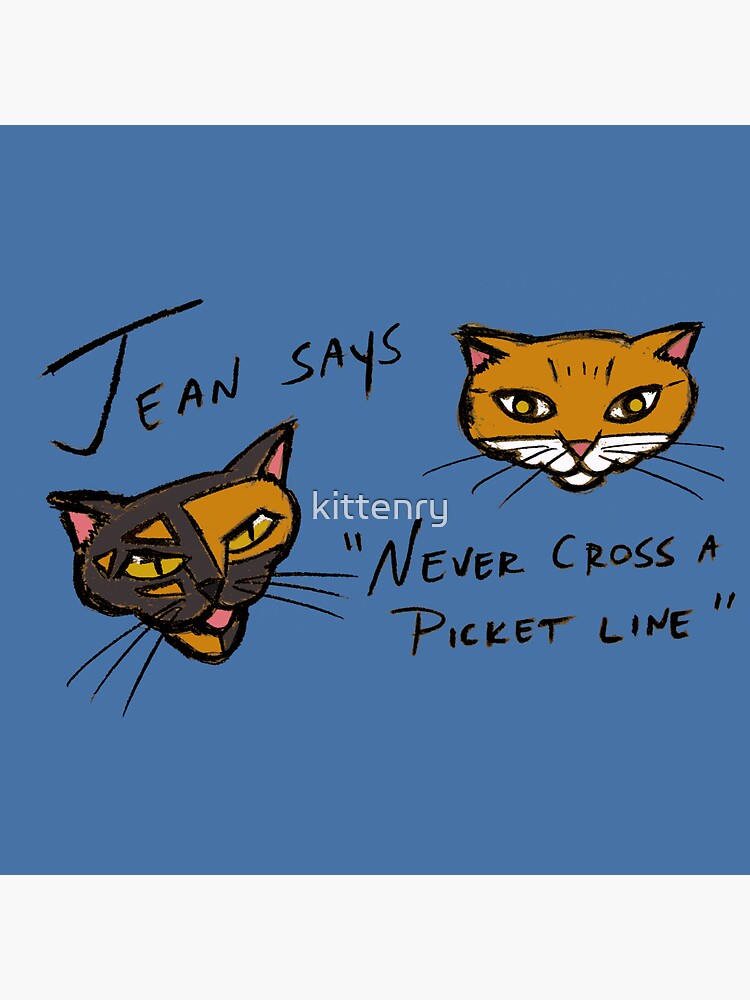The image is an illustration, possibly a poster, featuring two cartoon cat faces against a blue background that is slightly darker than sky blue. There is white letterboxing at the top and bottom of the image. 

On the left is a simplified depiction of a tortoiseshell cat with black and orange fur. This cat has yellow, oval-shaped eyes with vertical slit pupils, a black nose, and pink triangular ears. It also has black and orange markings, with distinct orange triangles around its right eye and a pink tongue visible in its open mouth. The fur around its neck is divided into orange on the left side and black on the right.

On the right is an orange cat with a white muzzle area, a pink nose, and similar pink triangular ears. Its eyes are yellow with visible whites, giving it a lively expression. This cat also has big black eyes with yellow dots in the center and six whiskers—three on each side of its face.

Text elements in the illustration include "Gene says" in black, handwritten-style text positioned above the tortoiseshell cat, and "Never cross a picket line," also in handwritten black text, placed below the orange cat. In the center of the image, there is a small watermark in white regular text that reads "kittenry."

The overall sketchy and scratchy drawing style of the cats adds a charming, cute aesthetic to the illustration.